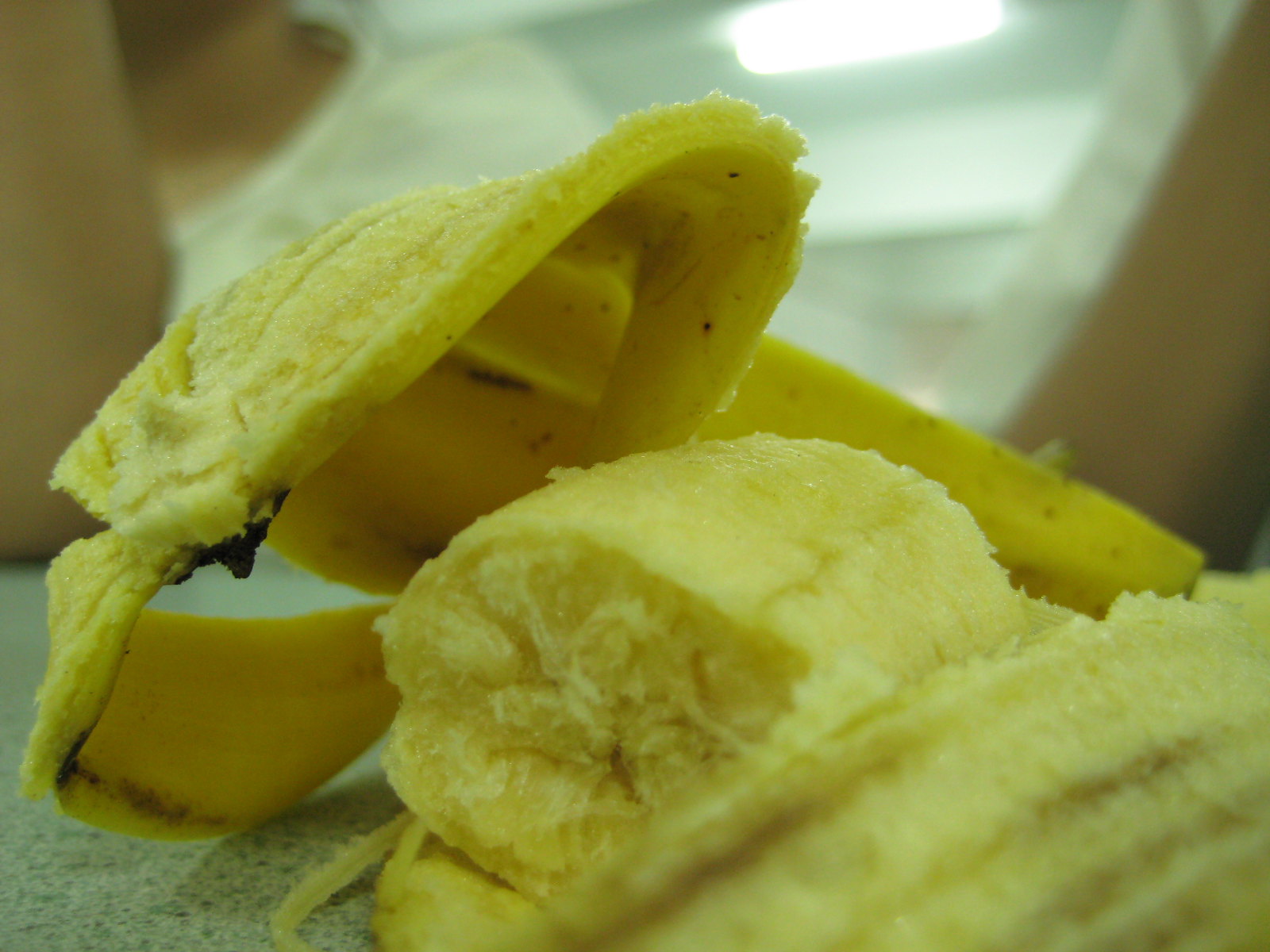An up-close photograph of a banana showcases its vibrant yellow peel, which is speckled with small brown spots and slightly folded over itself in a casual manner. The focus of the image is on the exposed, tender, and creamy yellow flesh of the banana. The background is artistically blurred, bringing attention to the detailed textures and colors of the fruit, highlighting its ripe and natural appearance.